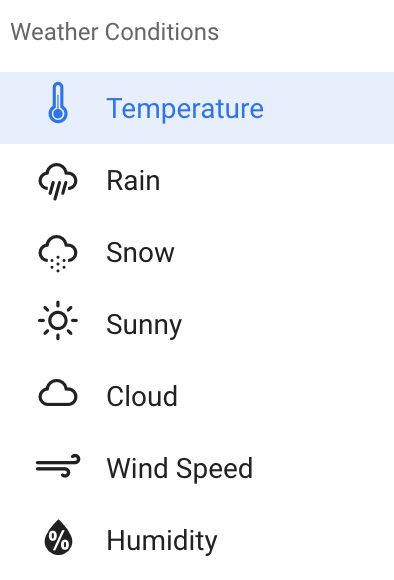A detailed close-up image of a phone screen displaying a weather application interface. At the top, in bold text, it reads "Weather Conditions." Directly below, a light blue rectangle with darker, royal blue text shows the current temperature, accompanied by a small thermometer icon on the left. 

Further down the screen, various weather conditions are illustrated with icons aligned to the left and their corresponding descriptions to the right. First, a rain cloud icon with diagonal lines depicting rain is labeled "Rain." Below it, a cloud icon with small gray dots represents "Snow." Following this, a circle with radiating lines symbolizing the sun is labeled as "Sunny." Next, a simple cloud drawing simply noted as "Cloud." Continuing down, two curved horizontal lines, the top one being longer than the bottom, indicate "Wind Speed."

Lastly, a black droplet icon contains a percentage sign inside, denoting "Humidity." This thoughtfully organized interface provides a comprehensive overview of various weather elements, each clearly represented with icons and labels.